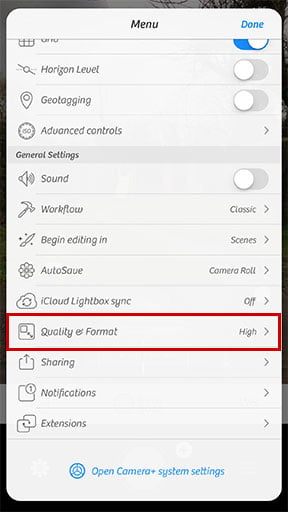The image is a screenshot from a mobile phone, displaying a settings menu overlay against a dark background. The top and bottom of the background are black, partially obstructed by the menu popup, which features a light gray to off-white color scheme. Centered at the top of the popup is the word "Menu" in black text with a capital M. On the right side, "Done" is written in bright blue text with a capital D.

Below, the screen details various settings and their statuses. The first setting is chosen as "On," though the specific option is partially obscured. Next, "Horizon level" and "Geotagging" are both turned off. Following these, "Advanced controls" appears, indicated by a right arrow on the right side.

The "General settings" section follows, specifying several options: "Sound" is turned off, "Workflow classic" has a right arrow, "Begin editing in" is marked with "Scenes" and another right arrow, "Autosave camera roll" also has a right arrow, and "iCloud white box sync" is off, accompanied by a right arrow.

Under the "Quality and format" section, "High" is highlighted with a red outline. Further down, settings for "Sharing," "Notifications," and "Extensions" are listed, each accompanied by a right arrow.

At the bottom of the menu, there is blue text reading "Open camera system settings."